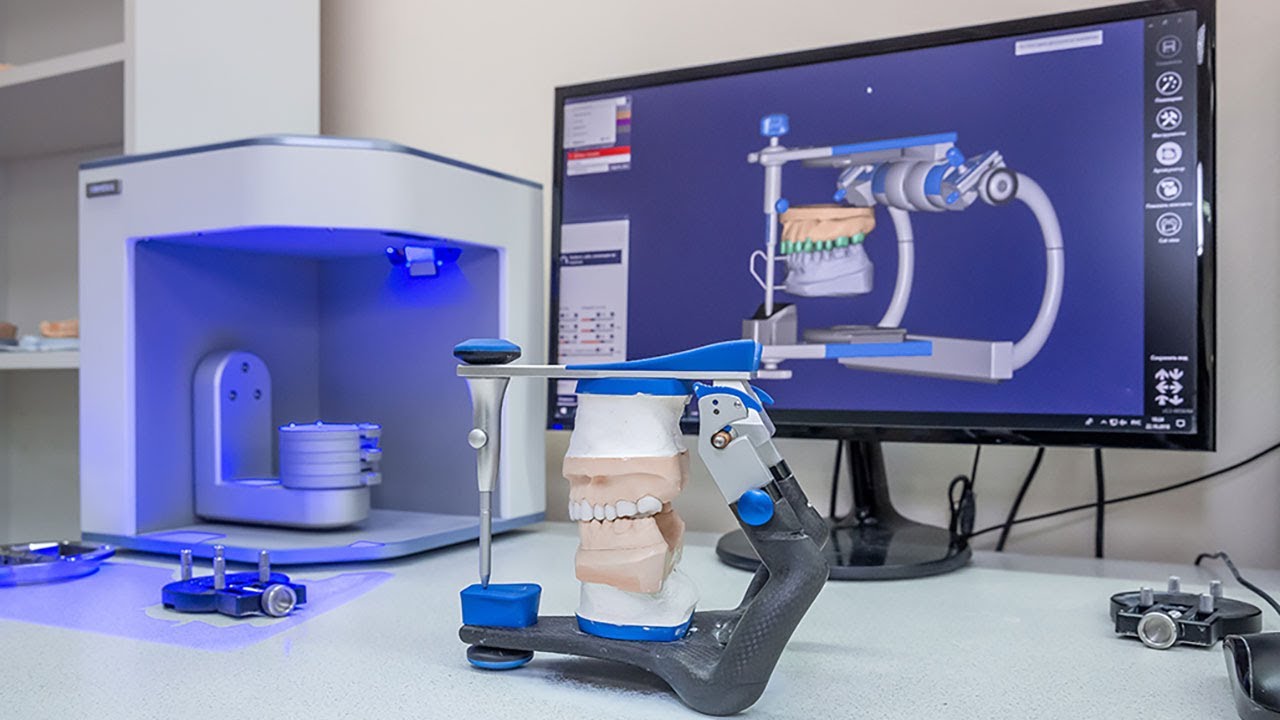The image depicts a detailed scene inside an orthodontic lab. Central to the image is a large black monitor displaying a 3D model of teeth, with various colors including blue, white, and gray. The screen also shows numerous pipes and text, though the words are unreadable. In the foreground, there is a physical clamp adorned with dentures, replicating the digital model seen on the monitor. This clamp features a mix of dark gray and blue components, with a long stick extending from the top to the bottom. 

To the left, there's a white shelving unit holding various items, and a blue, dollhouse-like square structure with its front cut out, illuminated by blue lighting. A round object sits on this blue structure, vaguely resembling a toilet but likely something else. Black light or infrared light equipment can be seen next to this setup. On the right side of the table, several gray and black devices are scattered, alongside cords running behind the monitor. The scene is awash with multiple colors, including varying shades of blue, gray, silver, off-white, and occasional touches of green and red, creating a highly technical and sterile atmosphere indicative of an indoor lab setting.